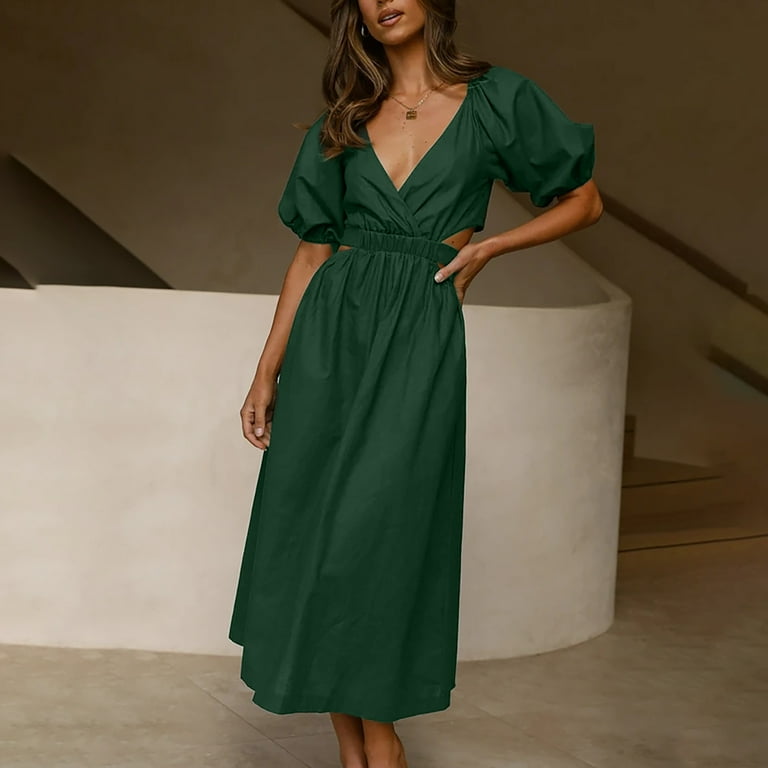In this color photograph, a tanned woman stands confidently in a modern foyer on a beige marble floor, in front of a white wall that transitions into a curved staircase with an outlined railing. She is modeling a green cutout dress with a deep V-neck, puffy sleeves ending at her elbows, and waist cutouts, which flows down to just above her ankles. Her left hand is placed on her hip while her right arm hangs by her side. She has long, slightly wavy brown hair, luscious lips, and accessorizes with a pretty pendant necklace and white-painted nails. The top half of her head, including her eyes, is cropped out of the frame, focusing the viewer’s attention on her ensemble and stance. The overall lighting is dim, adding a dramatic touch to the fashion-forward image.